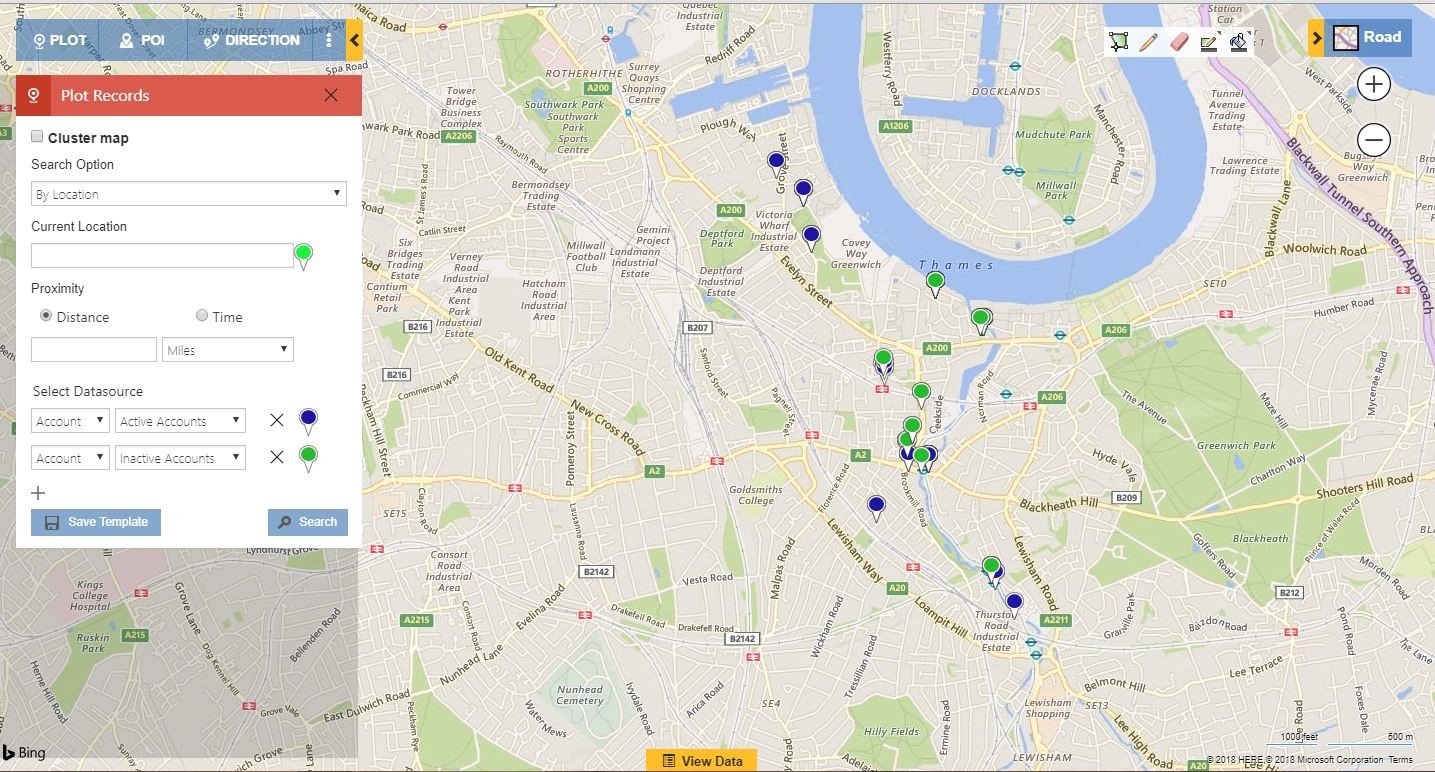A detailed digital map is displayed on the screen, showcasing various locations and landmarks. Predominantly, the background features a colorful map with different hues representing distinct areas; roads are highlighted in yellow, green marks represent land areas, and water bodies are colored in blue. Notable locations on the map include the Blackwall Tunnel Southern Approach, a discernible road. The River Thames, labeled clearly, meanders through the upper portion of the map, curving around the top and providing a distinct blue arc.

Specific neighborhood names like Docklands are visible, as well as parks such as Mudchute Park and Rotherhithe South Park. Major roads including Old Kent Road and New Cross Road can be identified. 

At the top of the screen, the heading "Plot Records" is visible, suggesting the mapping service or company in use. Various checkboxes are present, offering options for "Cluster Map", "Search Options", "Current Location", and "Proximity". Around the map interface, there are tools such as pencils and erasers, along with a box labeled "Road". Additionally, zoom control options are available, with plus and minus symbols for zooming in and out, respectively.

The interface also features pins that can be placed on the map, indicating points of interest or specific locations. The overall layout of the map is user-friendly, equipped with interactive tools for detailed navigation and customization.